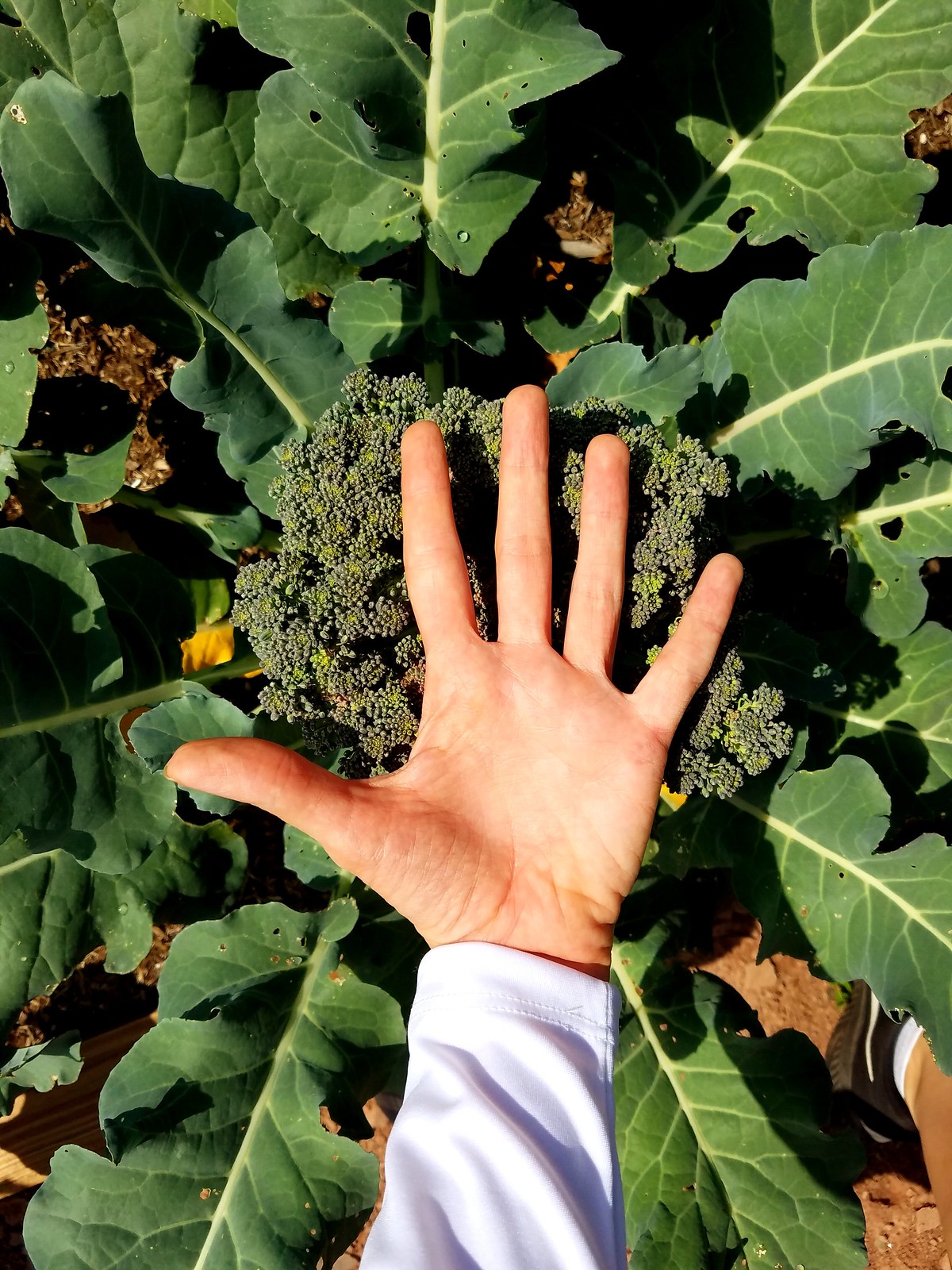In this detailed outdoor photograph, a man's left hand takes center stage, held palm-up amidst the lush greenery. He is wearing a white long-sleeved shirt that ripples slightly with wrinkles. The hand appears to float over a large, dark green plant that strongly resembles broccoli in texture and structure, almost encompassing the size of the hand itself. Radiating from beneath this central broccoli-like feature are wide, wavy leaves with conspicuous veins, some of which display touches of yellow and brown, suggesting varied sunlight exposure. The overall composition captures the contrast between the white shirt and various hues of green leaves, set against the natural backdrop of a garden. Sunlight bathes the scene, highlighting the intricate details of both the plant and the hand.